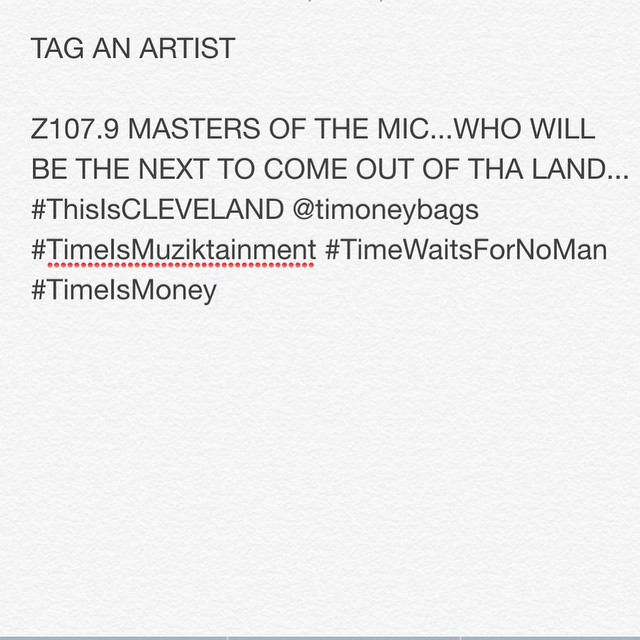The image features black text on a white background, which could either be a screen view or printed on paper. At the top, in capitalized letters, it prominently states, "TAG AN ARTIST." Below that, also in capital letters, the text reads, "Z107.9, MASTERS OF THE MIC... WHO WILL BE THE NEXT TO COME OUT OF THE LAND...". Following this, the text includes several hashtags and handles: "#ThisIsCleveland," "@TiMoneyBags," "#TimeIsMusikTainment" (spelled as M-U-Z-I-K tainment), "#TimeWaitsForNoMan," and "#TimeIsMoney." The hashtag "TimeIsMusicTainment" appears to be underlined in red dots. The text is straightforward and clearly laid out for promotional purposes, perhaps related to a music event or contest.